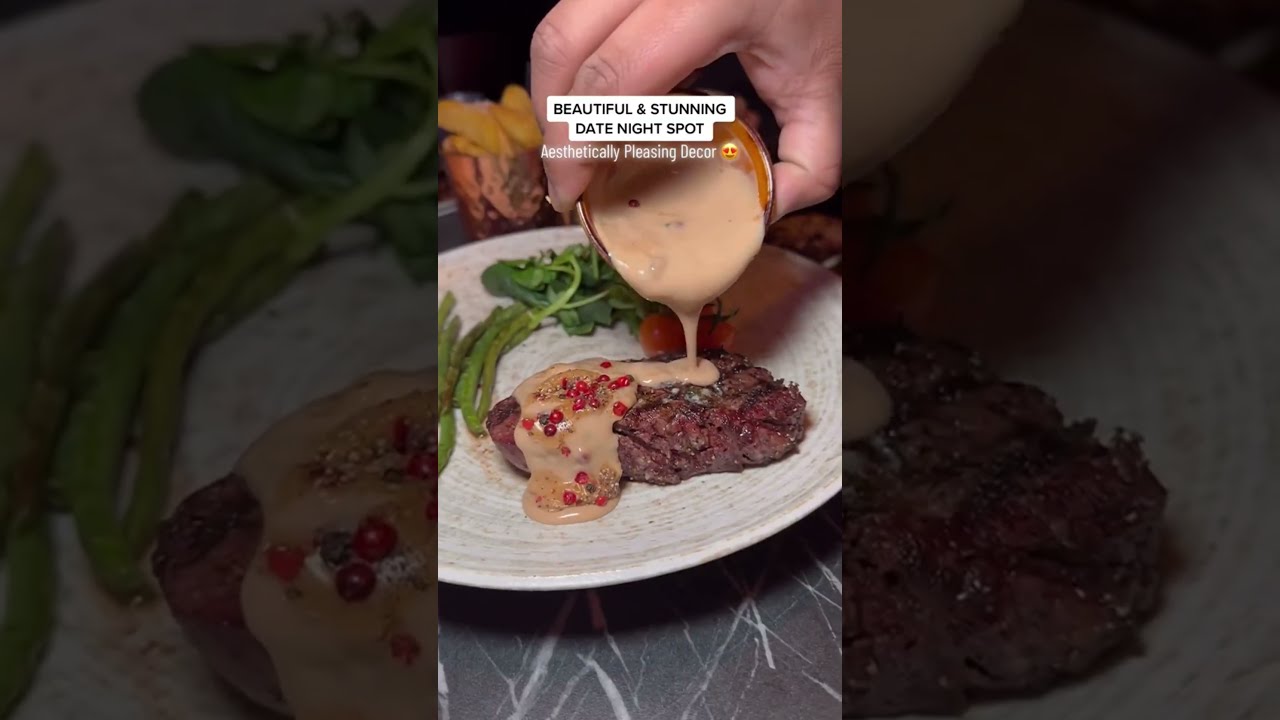A beautifully composed vertical cell phone photograph captures a delicious moment of a right hand pouring a tan, fish egg-laden sauce over a perfectly cooked steak, accompanied by asparagus, cherry tomatoes, and other greens arranged on a light tan plate. The scene is set on a sleek black and white stone countertop. Enhancing the visual appeal, the background consists of faded, zoomed-in fragments of the main image, providing a darkened and artistic frame on the left and right sides. Overlaying this sumptuous food scene, white text in rectangles declares it as a "Beautiful and stunning date night spot," while below, more text reads "Aesthetically pleasing decor," next to a heart-eyed emoji, emphasizing the charm and allure of the setting.